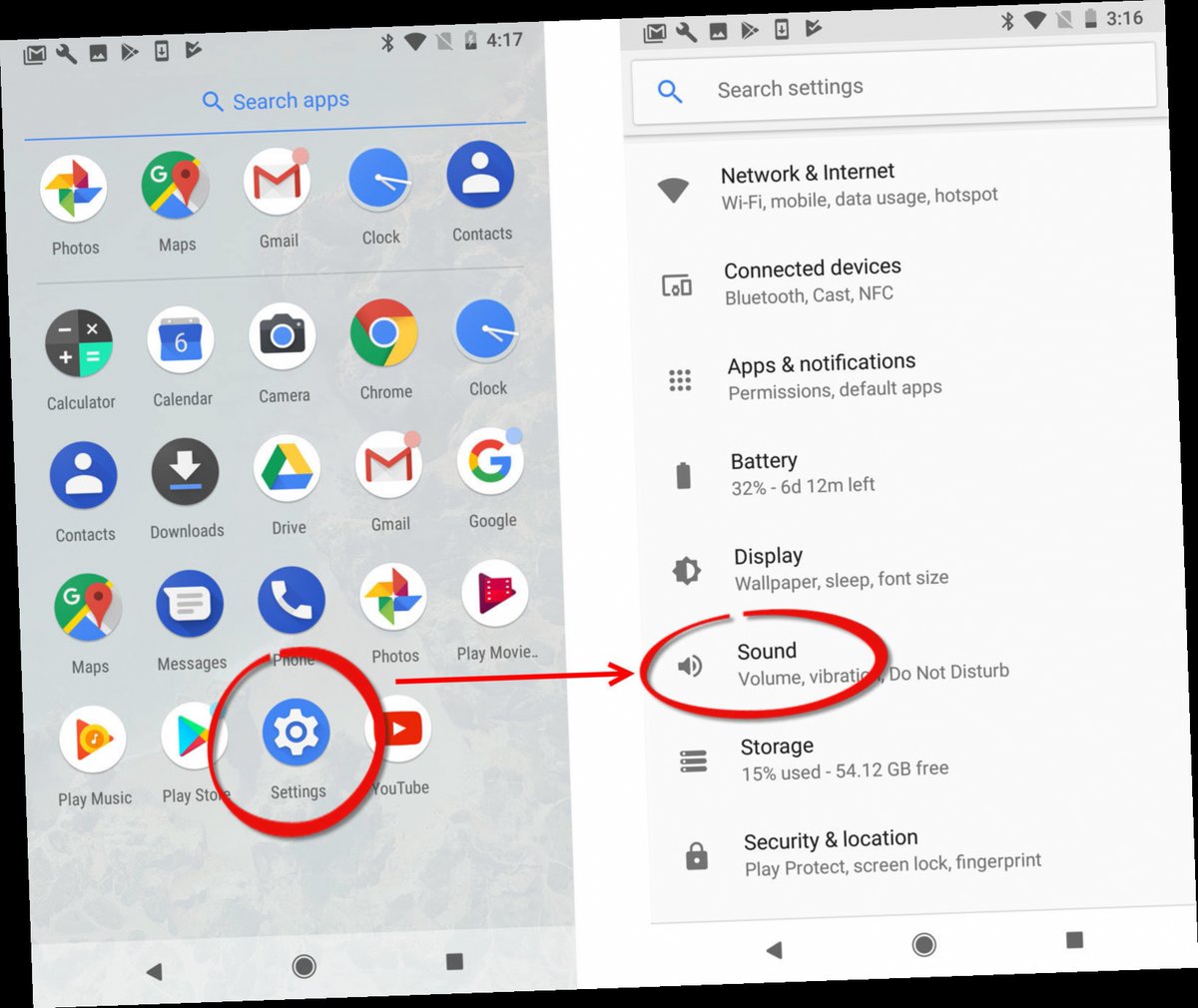This image features two side-by-side screenshots showcasing different sections of a smartphone's settings interface. Both screenshots exhibit a similar layout with menu options along the left side and top of the screen. Visible at the top are icons indicating the time (4:17), Bluetooth status, Wi-Fi connectivity, and battery life.

The screenshot on the left displays a row of commonly accessed apps, including Photos, Maps, Google, Gmail, Clock, and Contacts at the top, followed by four additional rows containing five different icons each, presumably for various application and system settings. 

The right screenshot mirrors the menu options present in the left image, featuring the same "Search Apps" and "Search Settings" bars at the top. It mainly focuses on the broader categories in the device's settings menu. These categories are listed as follows:
1. Network and Internet
2. Connected Devices
3. Apps and Notifications
4. Battery
5. Display
6. Sound
7. Storage
8. Security and Location

In this composite image, two particular settings are highlighted. The "Settings" option in the left screenshot and the "Sound" option in the right screenshot are both circled in red, with a red arrow drawn pointing towards them, indicating a focus or relevance to these sections in the contexts depicted.